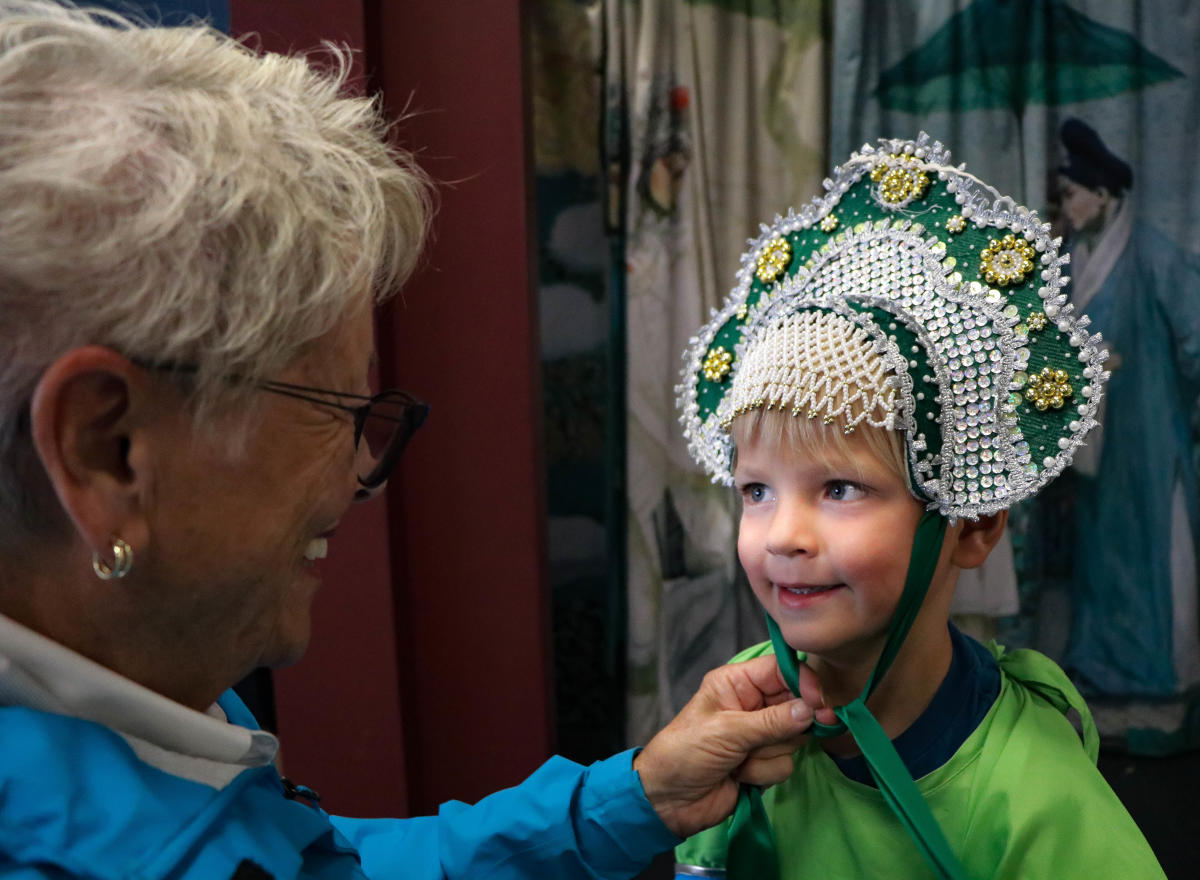In this detailed horizontal color photograph, an elderly woman with short white hair, dark glasses, and a silver earring is seen on the left side. She's wearing a bright blue shirt with a white collar and is smiling warmly as she affixes an ornate headdress to a young boy standing before her. Her left arm is extended, and she is tying the headpiece under the boy's chin with a dark green ribbon. The boy, who has bright blonde bangs and rosy cheeks, is also smiling up at her. He is dressed in a distinctive costume that includes a green smock over a blue crew neck shirt. 

The headdress, resplendent in its detail, features intricate beadwork, green and white bands, pearls, golden spheres, baubles, and bangles, with ornate stringing of beads adorning the forehead. Behind them, a tapestry or drape depicting a figure in a robe holding a green umbrella adds an additional layer of cultural richness to the scene, indicating that they might be preparing for a traditional or cultural event. The shared smiles and engaged interaction between the woman and the boy highlight a moment of tender connection during a festive preparation.